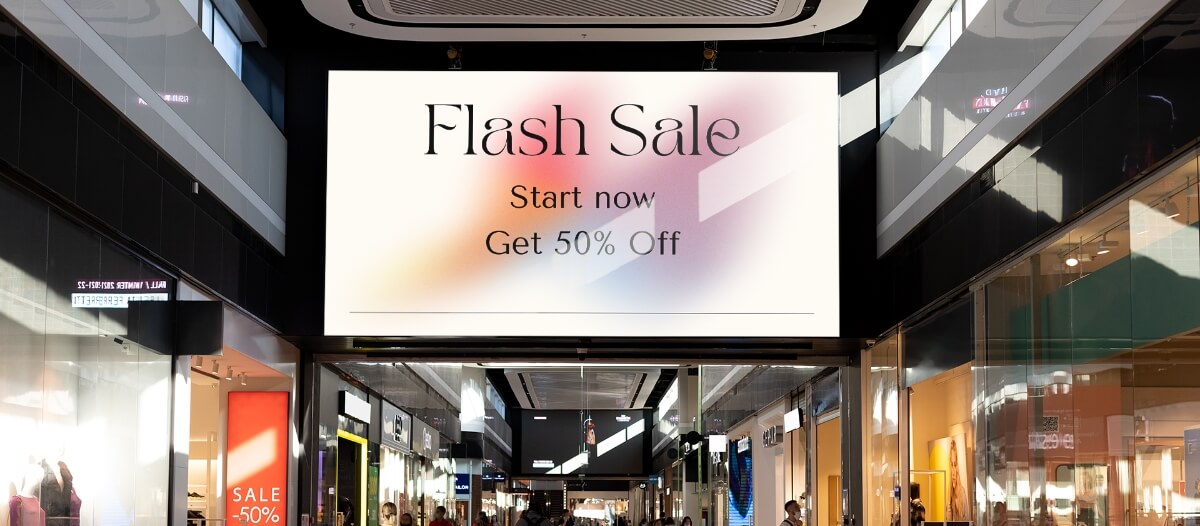The photo captures an indoor view of a bustling shopping mall with a high ceiling and glass-paneled store fronts on either side of a main corridor. Prominent in the frame is a ceiling-mounted sign that reads "Flash Sale, Start Now, Get 50% Off" in black text on a background adorned with pink and orange squiggles. Below this sign, the tops of shoppers' heads can be seen as they wander through the mall. Reflections of lights and colorful sale signs, including a prominent red sign with "Sale 50% Off" in white letters, are visible in the glass windows of the stores, which feature mannequins displaying various clothing items. The ceiling, decorated in shades of gray with horizontal gray columns, further emphasizes the modern design of the mall.